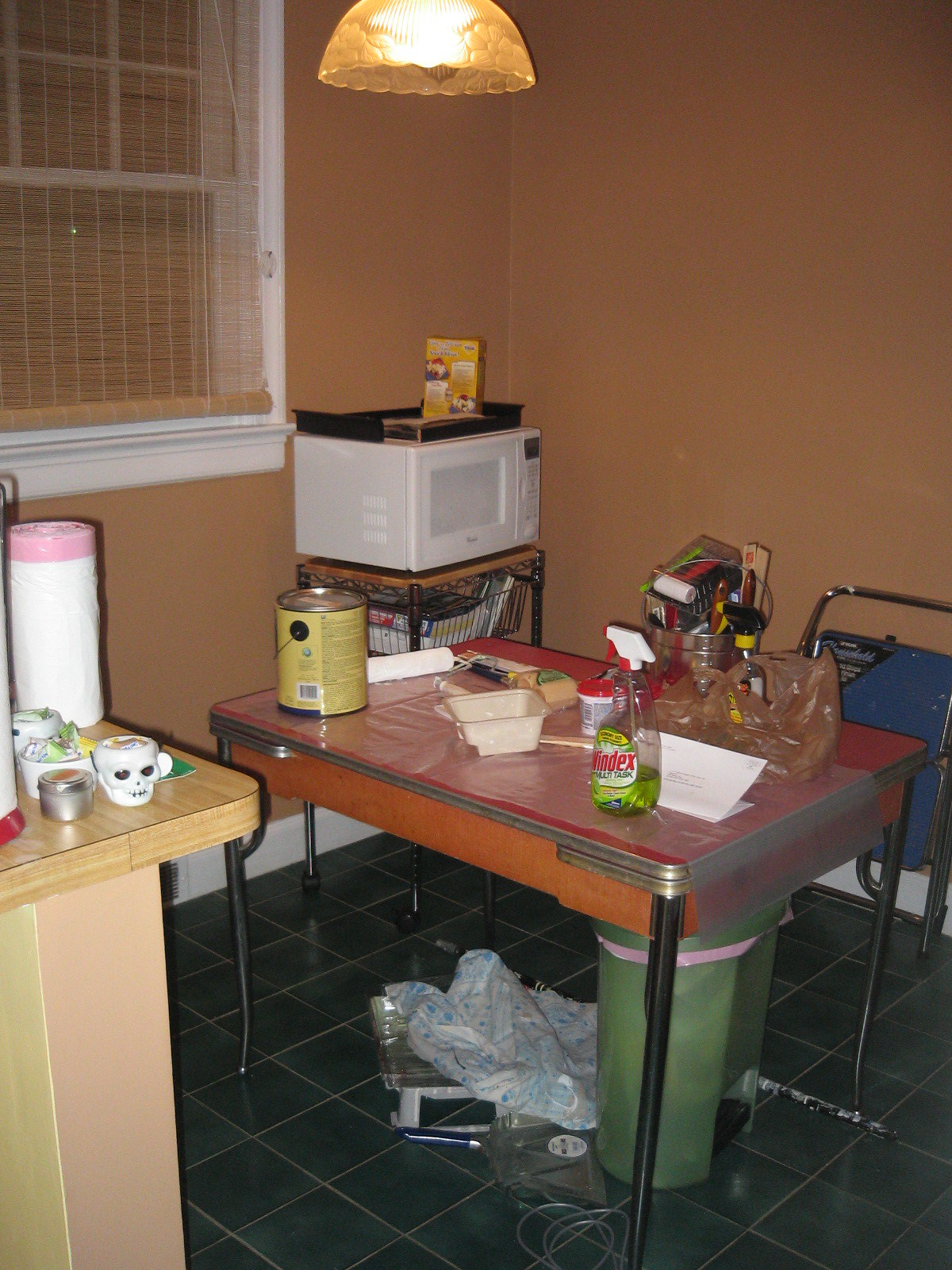A well-used kitchen is depicted in this photograph, framed by warm brown walls. A prominent domed glass light fixture, casting a yellowish glow, hangs from the ceiling, reflecting light off its smooth surface. At the back of the kitchen, a window with a grid pattern on its top section consisting of four square panes stands partially concealed by a roll-up bamboo shade. The scene outside the window is dark, indicating that the image was taken at night.

Situated against the back wall, a simple white microwave rests atop a small, black wire cart with a brown top. On the microwave, a black bin contains various items. In the center of the room, a small, vintage dining table with a brown base, red top, and metal legs is visible. Atop this table, a paint can sits beside a Windex bottle and a piece of drop cloth, suggesting an ongoing renovation or cleaning project. Scattered supplies are strewn across the black tile floor, contributing to the overall cluttered atmosphere. A green garbage can, partially hidden, is tucked underneath the dining table.